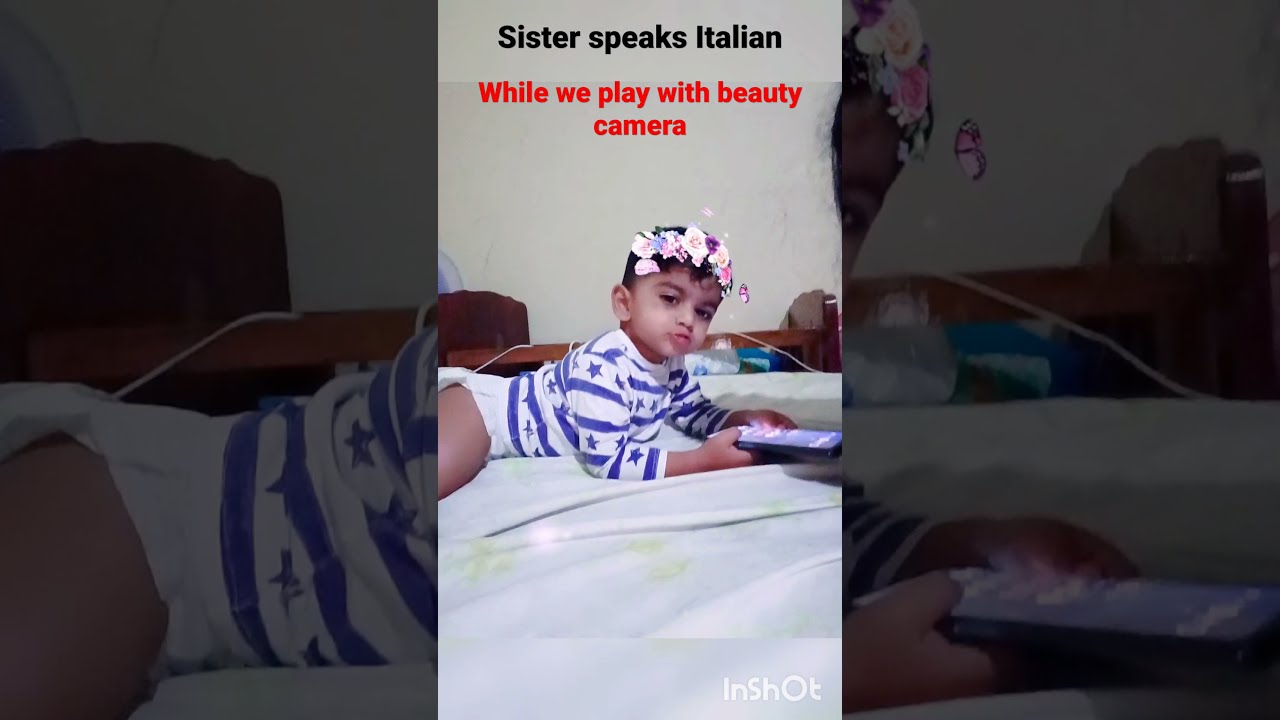The image captures a baby, approximately 3-4 years old, laying on a bed and looking at a cell phone. The baby is dressed in a white top adorned with blue stars and wearing a diaper. He has short black hair and is decorated with a Snapchat filter that places a flower headband around his head. The background reveals a plain white wall. Overlaying the image is a caption in black text at the top that reads, "Sister speaks Italian," followed by red text stating, "While we play with beauty camera." A watermark at the bottom right corner says "InShot."